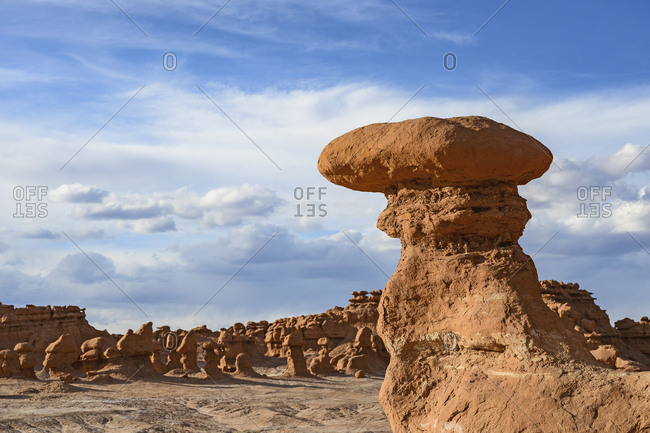The image depicts a vast, deserted area resembling the Grand Canyon, featuring numerous jagged rock formations and plateaus spread across the landscape, primarily made of red clay, stone, and some shades of off-red and brown. Dominating the right side of the image is a particularly tall rock structure with a substantial, flat boulder precariously perched atop a jagged stalk, extending from the lower right corner to above the midpoint. The lower portion of the scene contains ground composed of stone and clay, fading into sand towards the left. In the distance, a line of similarly jagged rocky structures creates an impressive backdrop.

The upper two-thirds of the rectangular image is filled with a blue sky dotted with various clouds—some fluffy, some wispy—predominantly gathering in the middle part of the sky, with fewer at the top. 

Overlaying the image is a grid-like watermark, displaying the word "offset" multiple times. The first instance is positioned on the far left, with "off" written normally and "set" directly beneath it but rotated 180 degrees, resulting in the characters 'T', 'E', and 'S' appearing upside down. Similarly, "offset" appears again just below the left edge of the flat boulder and once more to the right of the flat boulder, all rotated and positioned at 45-degree angles. The image is bright, suggesting it is daytime, though the sun is not visible.